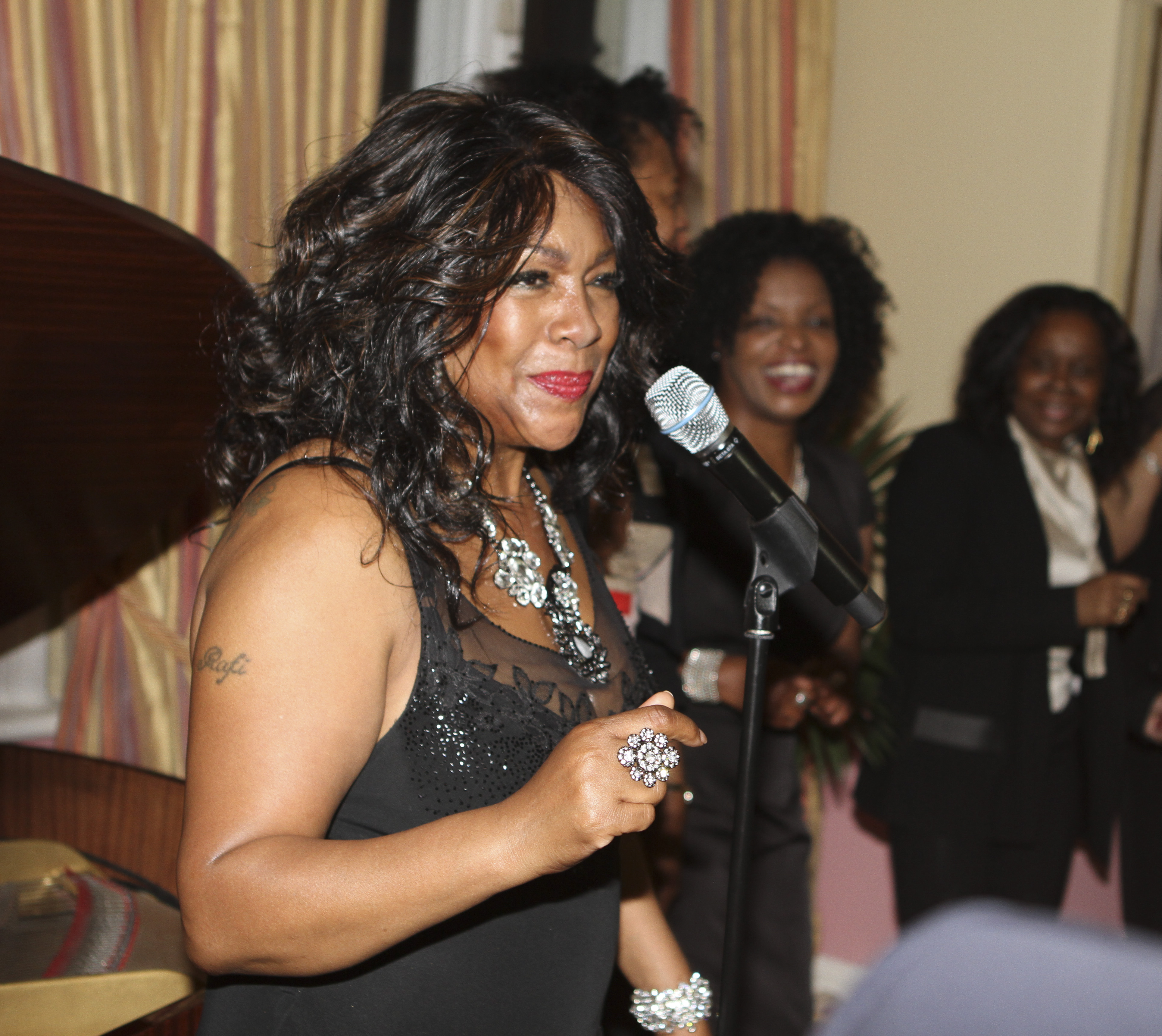This indoor photograph captures a vibrant scene centered around a woman who appears to be singing into a black microphone with a silver rounded top, held on a black stand. She is adorned in a sleeveless black dress with thin straps, and her ensemble is complemented by an eye-catching array of silver jewelry: a necklace with floral ornaments, a shiny wristband, and a large flower-shaped ring. Red lipstick adds a striking touch to her look. The woman, who has shoulder-length brown hair and a visible tattoo on her left arm reading "Rafi", seems to be commanding the attention of her lively audience. Behind her, a tan-colored wall with draped striped curtains sets the backdrop for multiple people, all wearing black, who appear to be either dancing, clapping, or singing along. Among them, some are dressed in open jackets and dresses, contributing to the festive or ceremonious atmosphere that suggests the scene could be a party, gathering, or performance. Additionally, a raised section of a grand piano is subtly visible on the left, hinting at musical accompaniment for this engaging performance.